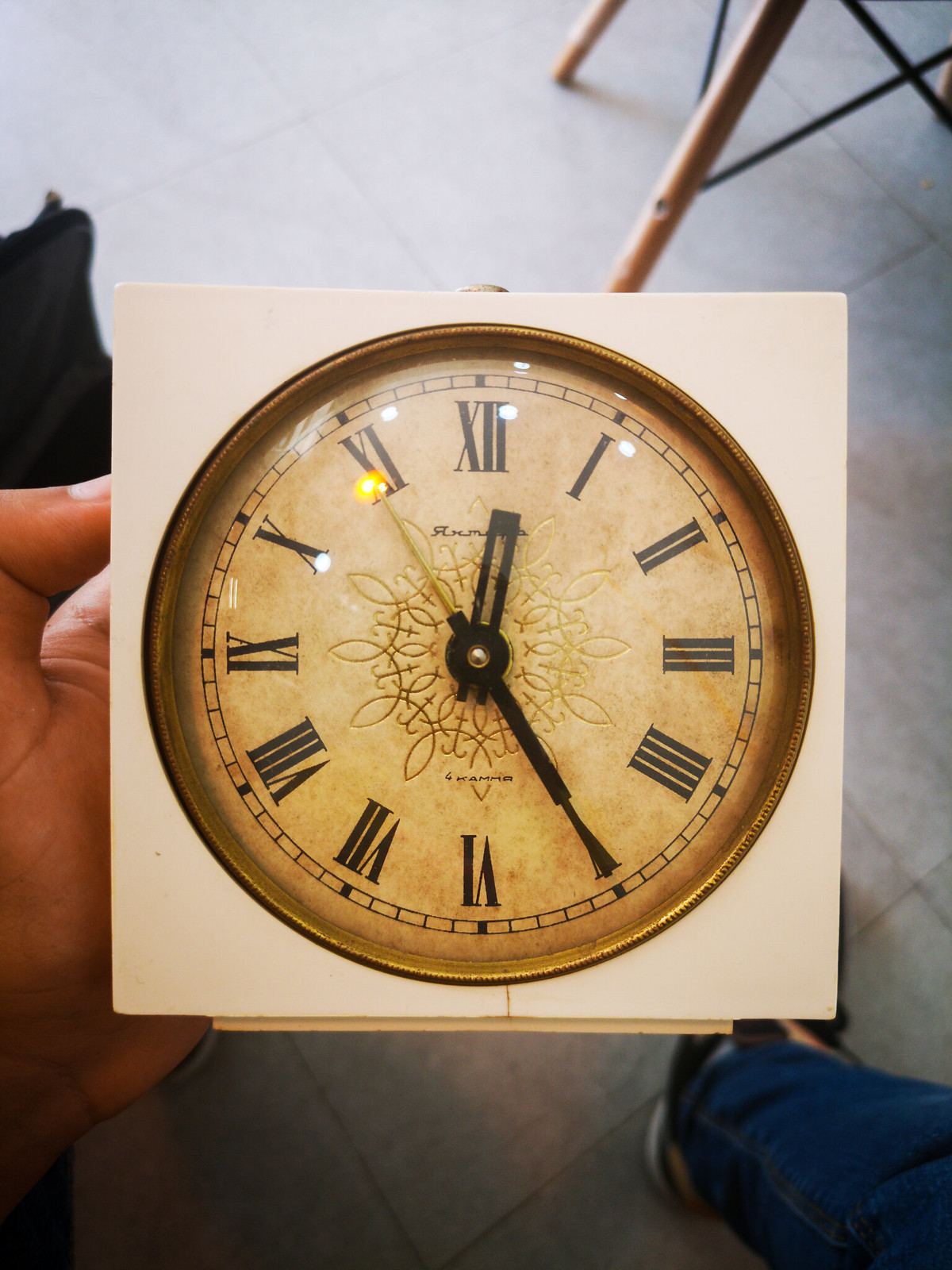A person is standing on a light gray tile floor, holding a clock in their left hand. They are wearing blue skinny-fit jeans, and a partial view of their shoe is visible, though mostly obscured by the clock. The clock is positioned centrally in the photograph and is enclosed in a white frame. It features a beige-gold clock face with Roman numerals and black hour and minute hands, indicating the time is approximately 12:25. In the upper right corner, the legs of a chair or stool are faintly visible. The person’s left hand extends into the frame from the left side, supporting the clock.